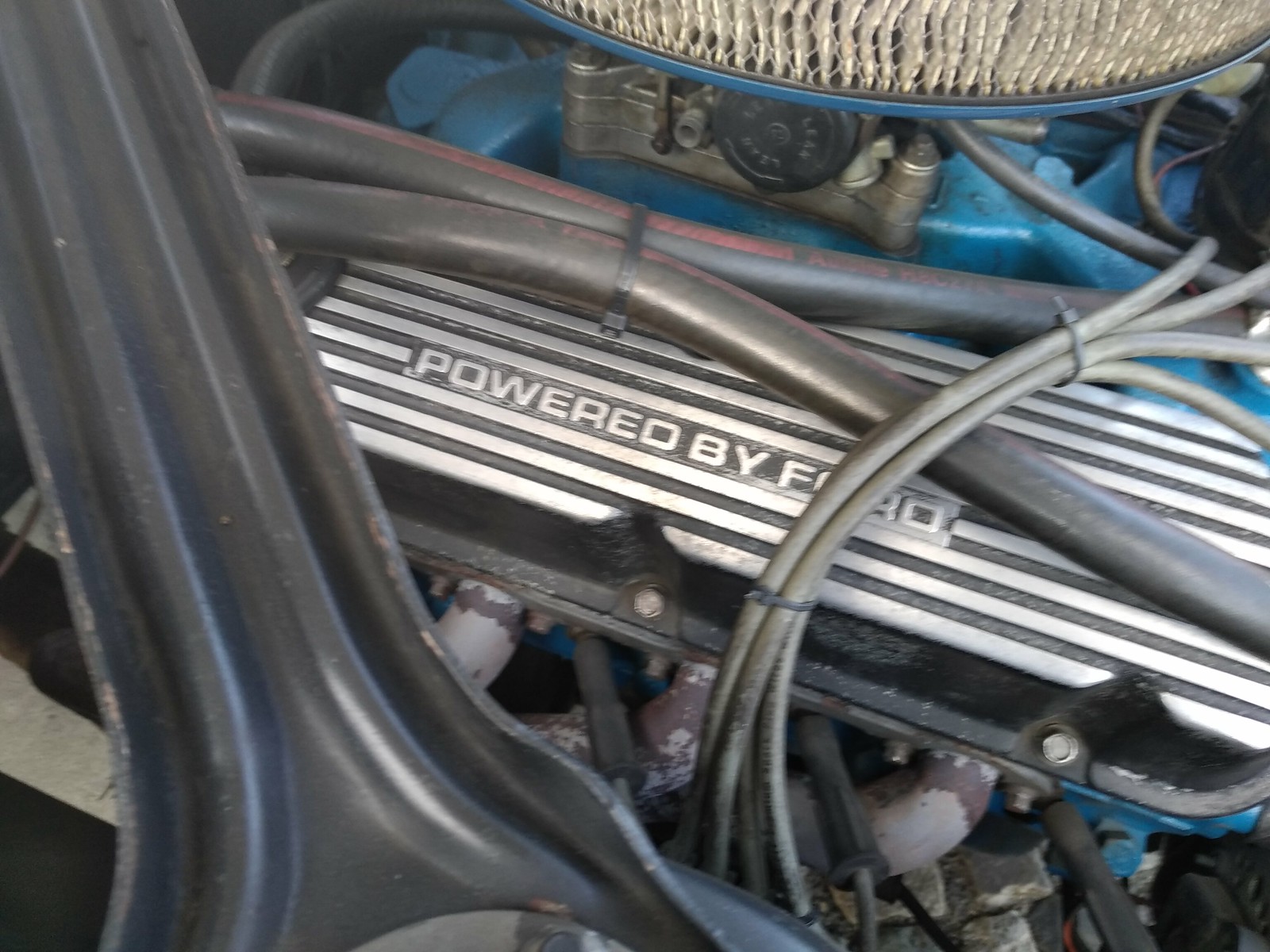This detailed photo captures the interior of what appears to be an older vehicle's engine compartment, prominently featuring a long metal piece in the center that reads "Powered by Ford" in white text. Surrounding this, a complex network of tubing and wiring is evident, including several thick, clamped tubes that run horizontally from left to right. These tubes are intertwined with smaller gray wires and tubing, some of which extend from the bottom and likely connect to an older-style air filter positioned at the top right. This air filter, which has a blue-painted underside, adds to the vintage feel of the engine. A large metal piece partially obscures the left side of the image, further adding to the cluttered mechanical environment filled with various metal parts, including what seem to be spark plugs and a carburetor. The lower part of the image reveals a grimy and gritty texture, reinforcing the impression of an aged and well-used engine compartment.